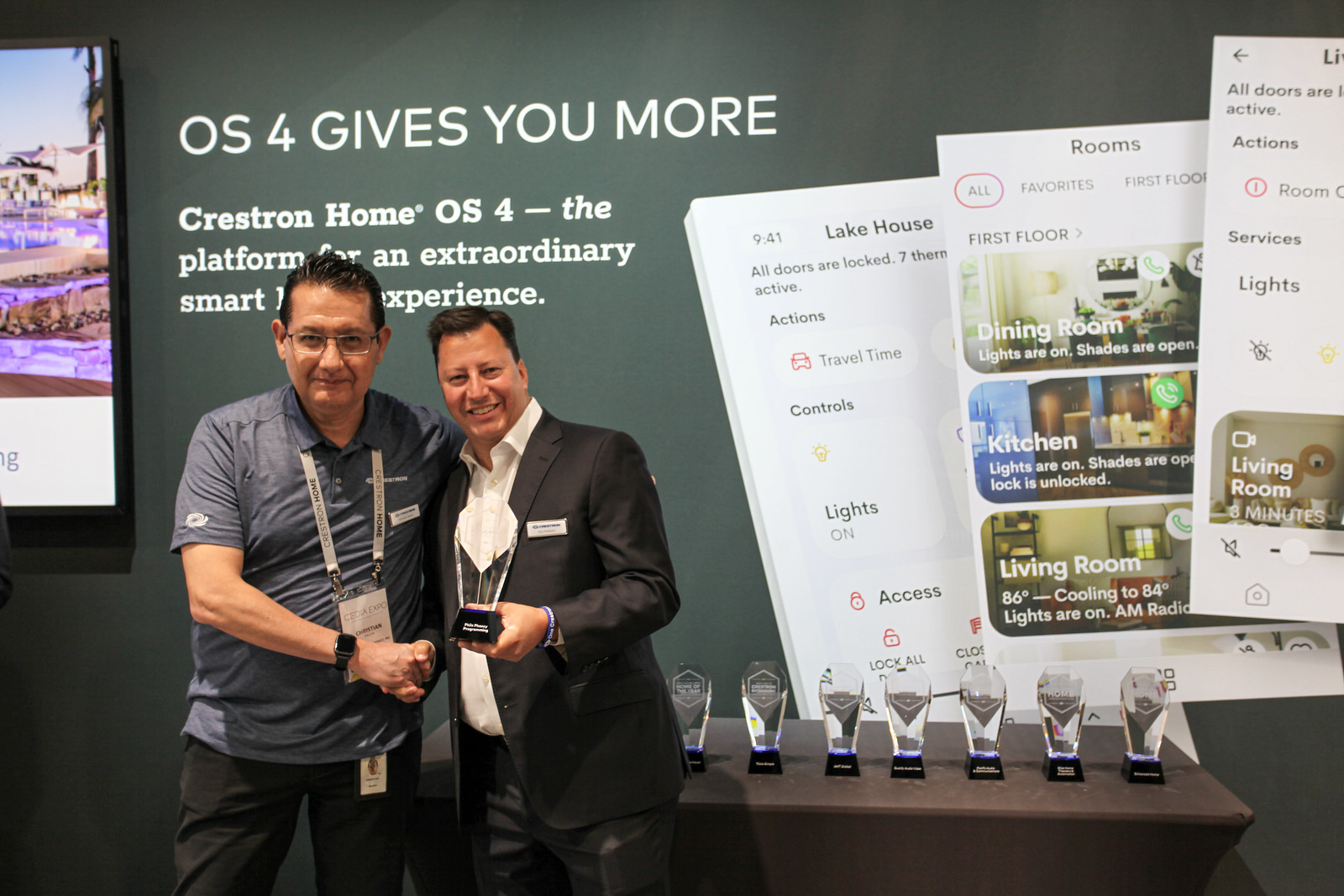In this image, two men are shaking hands in front of a backdrop that prominently features the slogan "OS4, the platform for extraordinary smart performance." The man on the left, dressed in a gray polo shirt, glasses, and a lanyard with a plaque displaying his information, wears a watch on his right hand. His counterpart on the right is adorned in a black suit with a white shirt, smiling brightly as he holds an award in his left hand. Both men are framed by a dark green wall that showcases seven trophies on a table to their right, with the eighth trophy being held by the man in the suit. The background also contains images resembling an Airbnb listing for a lake house. This celebratory scene exudes a sense of achievement and recognition, captured in the moment of receiving accolades.